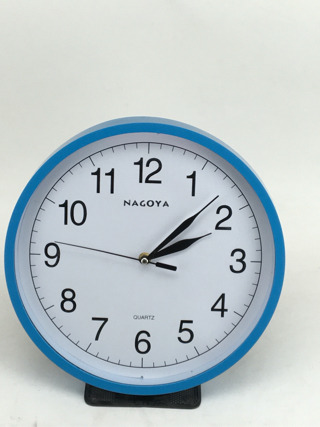A detailed view of a white Nagoya-branded clock set against a stark white background. The clock face is encased in a periwinkle blue plastic frame, contrasting sharply against the minimalist backdrop. The clock hands and the numerals, rendered in a standard black font, indicate the time as approximately 2:08, close to 2:09. The base of the clock is black, providing a visual anchor. A subtle drop shadow cast beneath the clock adds depth to the otherwise clean and uncluttered composition. The clock is positioned slightly off-center to the left, adding a touch of asymmetry to the image.